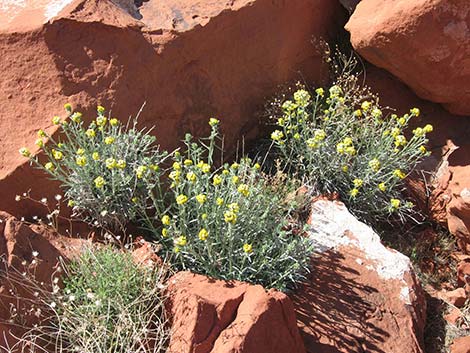On a hot, sunny day, this image captures a rugged, desert landscape marked by clay-colored, light brownish rocks. Nestled within the cracks and crevices of these rocks, thriving against the dry backdrop, are several clusters of resilient greenery. These shrubs and weeds are adorned with small, yellowish flowers, lending a contrasting burst of color to the scene. Additionally, there are hints of tiny white flowers scattered intermittently among the foliage. The rocky surface shows signs of wear with white powdery scrapings, and scattered rubble can be observed in the background. Despite the harsh, arid conditions, the flora manages to survive and add life to this otherwise barren setting.